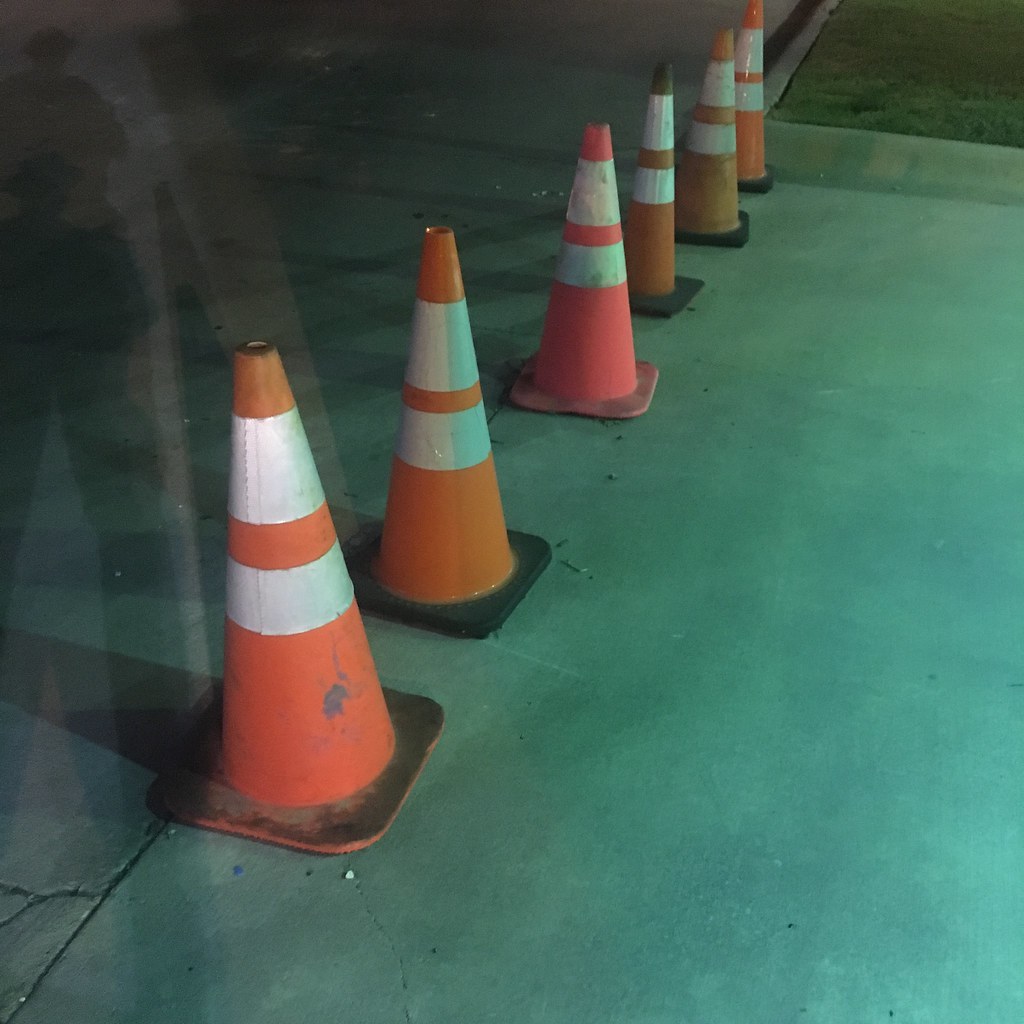The photograph captures a scene featuring six traffic cones lined up in a row on a cracked and slightly dirty concrete surface. The traffic cones, varying in shades of orange, prominently display white reflective strips near their tops. Some of these cones appear weathered and dingy, with peeling orange and visible dirt, while others remain more pristine. In one corner of the image, a strip of green grass peeks into the frame, adding a touch of color contrast. A light reflection and the shadow of a person are also visible on the concrete, adding depth and a human element to the scene.